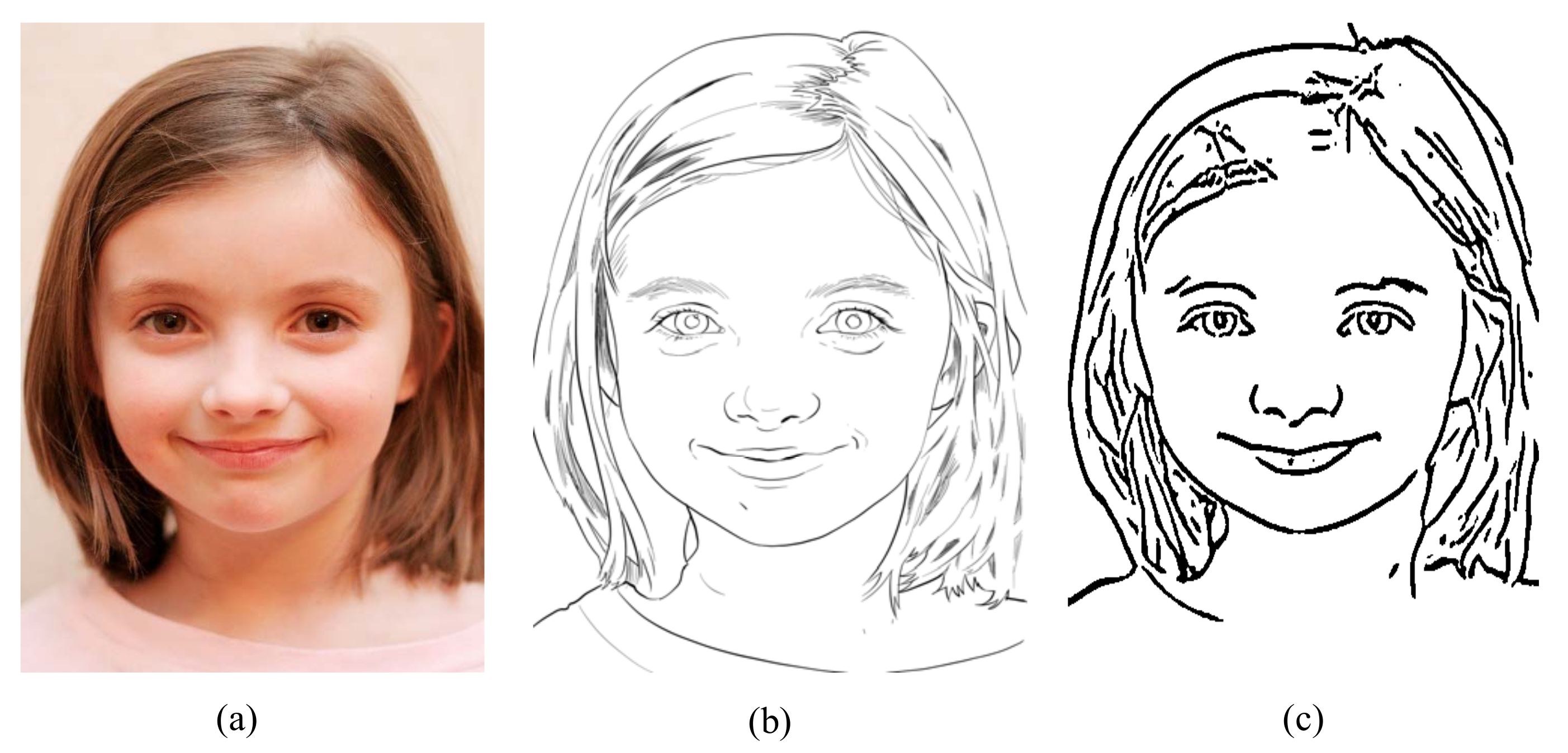The image is composed of three parts, labeled A, B, and C, from left to right. The first image (A) is a vibrant color photograph of a smiling young Caucasian girl with brown eyes and short, straight brown hair styled in a shoulder-length bob parted on the side. She is wearing a pink shirt and looking directly at the camera. The middle image (B) is a detailed black and white computerized outline sketch of the same girl, capturing the essence of the photograph but without any color. The third image (C) on the right is a rougher, less detailed hand-drawn sketch of the girl, also in black and white, emphasizing the progression from a highly detailed photograph to simpler artistic interpretations while retaining the fundamental features of her appearance.